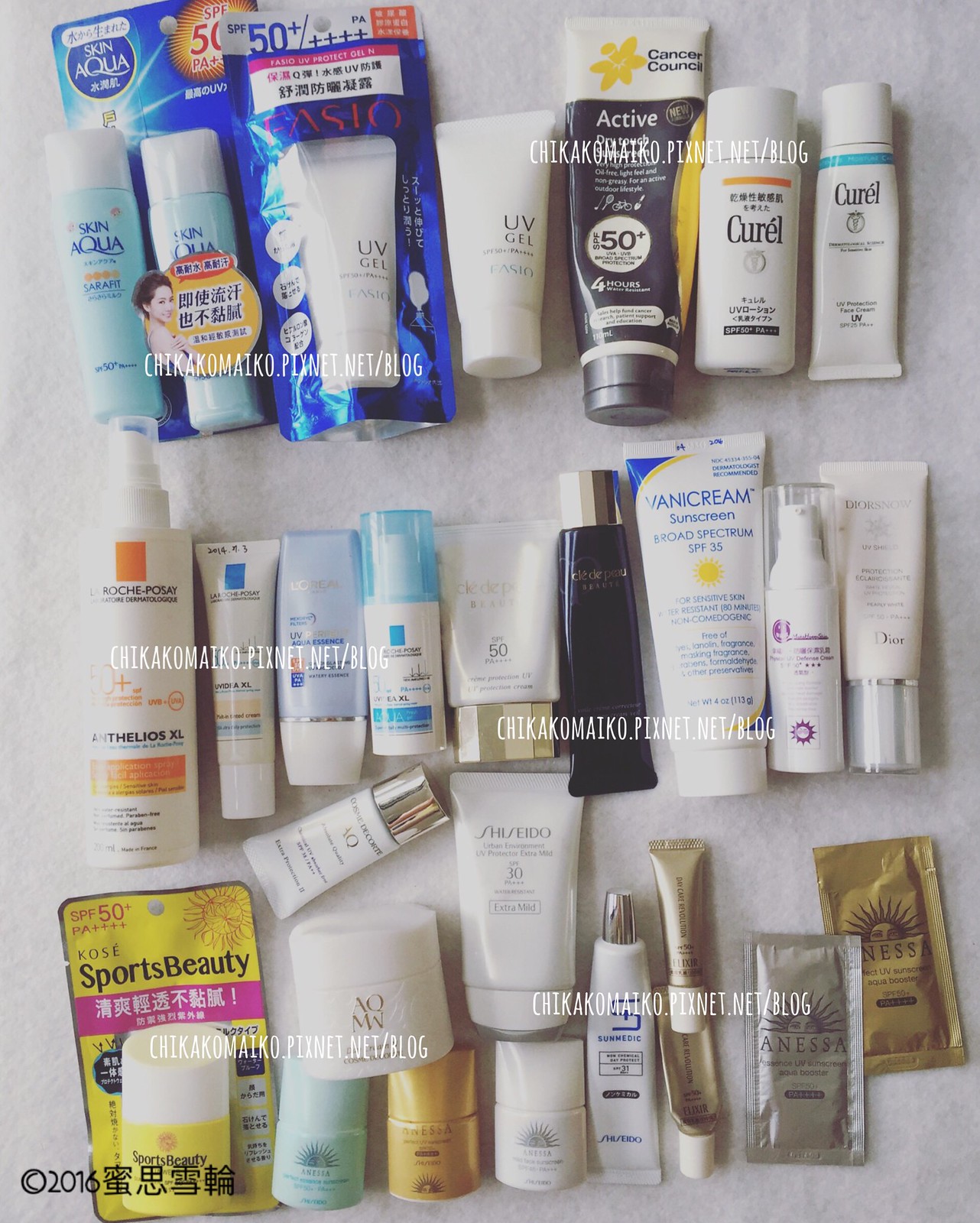This image showcases an extensive collection of beauty products meticulously arranged on a pristine white background. In the upper left corner, there are two packages of Skin Aqua sunscreen, each labeled "UV Gel" in white containers. Adjacent to these is another white and black container. Next in line is a cylindrical white container of Corel, followed by a tube of Corel.

Beneath this row, starting from the left, is a container from La Roche-Posay. This is followed by two partially readable tubes. Next is a container with a clear blue cap, followed by a white tube with a gold cap turned upside down. Beside it, there's a black tube with a gold cap turned right side up.

Further down, on the lower right side, is a patch labeled "Sports Beauty" with text in a foreign language, depicted in yellow and pink. Surrounding it are an additional nine varied beauty products, completing this diverse and well-organized display.